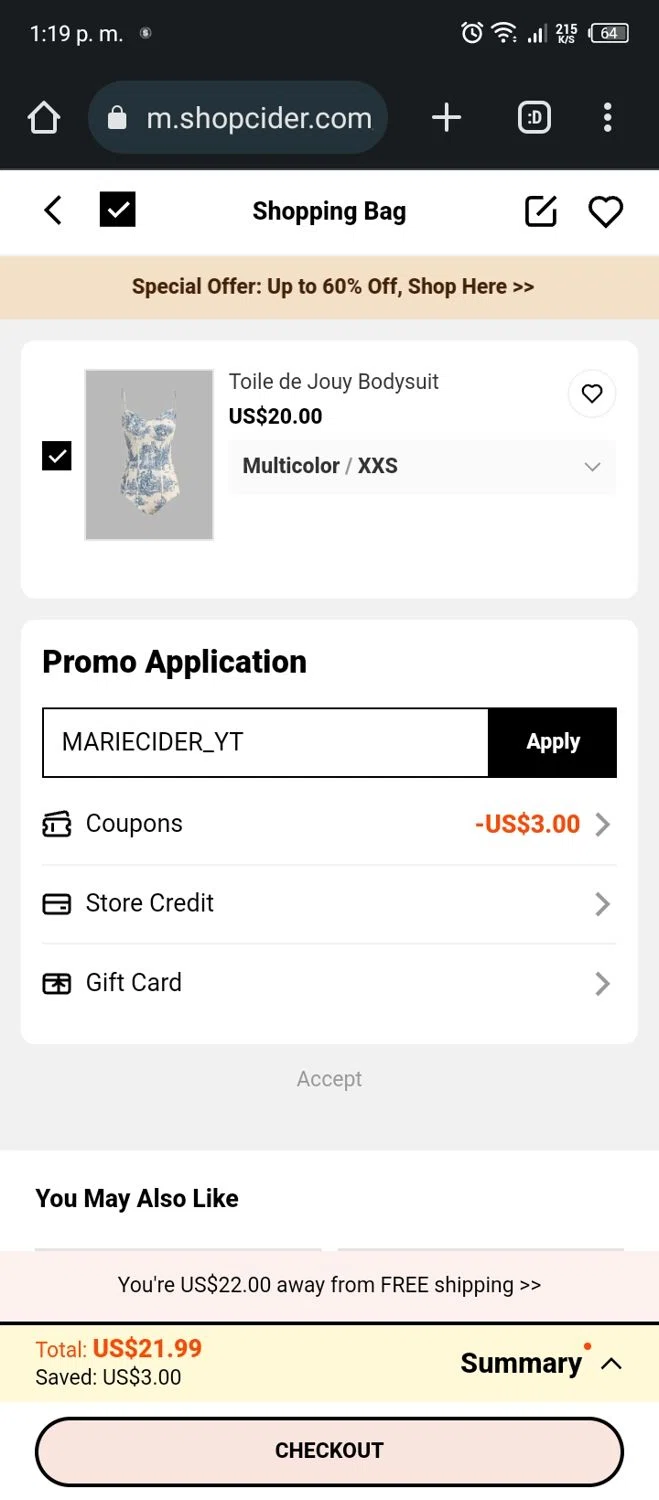A screenshot from a mobile device displays the shopping cart from the website m.shopsider.com. At the top, a brown tab advertises a special offer with discounts up to 60%. The shopping bag includes a "Toile de Joie" bodysuit listed for USD $20.00, described as being multi-colored and in an Extra Extra Small size. The bodysuit has a white background with intricate blue designs reminiscent of fine china.

Below the item details, there's a section for promo applications showing the code "MERRY CIDER_YT" in all capital letters, which results in a coupon discount of USD $3.00 highlighted in orange text. Additional sections for applying store credit and gift cards are visible beneath.

Further down, there's a light brown notification box informing the user that they are USD $22.00 away from qualifying for free shipping. A yellow box with orange text states the total cost as USD $21.99, alongside a black text note indicating a USD $3.00 saving. The order summary is presented to the right in black text.

At the very bottom, a light brown "Check Out" button encourages the user to finalize their purchase.